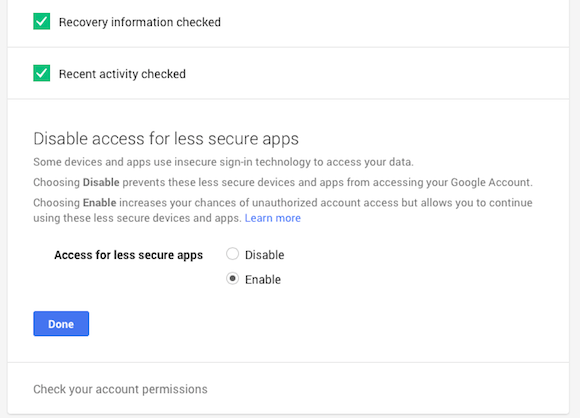A detailed screenshot depicts someone configuring their application settings, specifically within a Google platform. At the top, two green check marks indicate selected options: "Recovery Information Checked" and "Recent Activity Checked." Below these selections, a bold headline reads, "Disable access for less secure apps."

Accompanying the headline, a descriptive paragraph explains the potential risks and benefits associated with enabling or disabling access for less secure devices and applications. The text elaborates that some devices and apps utilize insecure sign-in technology to access user data. Choosing "Disable" prevents these less secure devices and apps from accessing the Google account, thereby enhancing security. Conversely, opting to "Enable" access increases the risk of unauthorized account access but allows continued use of less secure devices and apps.

A hyperlink labeled "learn more" is provided for additional information. Further down, a section titled "Access for less secure apps" offers two choices: "Disable" and "Enable." The "Enable" option is currently selected.

At the bottom, a prominent blue button labeled "Done" is displayed, with a final note below it instructing users to "Check Your Account Permissions." The screenshot has been cropped, leaving out some peripheral details. The interface is characterized by Google's typical white and blue color scheme, reinforcing its association with Google, despite the uncertain specific app being displayed.